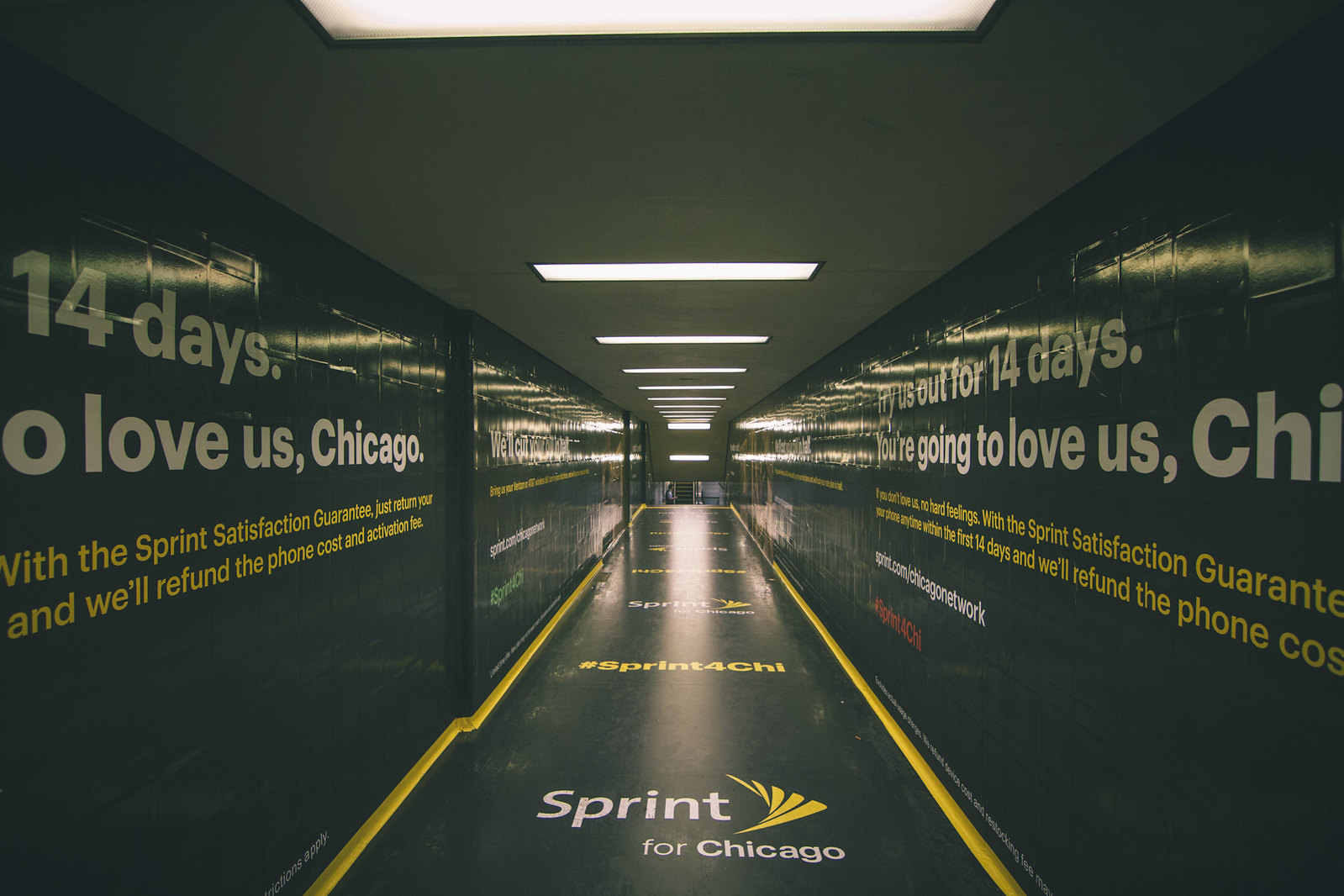The image depicts a dimly lit tunnel or hallway, most likely in a large building or an airport. The tunnel features dual walls lined with advertisements. On the left side, a large banner reads, "14 days to Love Us Chicago with the Sprint Satisfaction Guarantee. Just return your blank and we'll refund the phone cost and activation cost," with identical messaging mirrored on the right side. The floor bears the inscription "Sprint for Chicago" along with the Sprint logo, and further up there's a hashtag, "#SprintForChi." The ceiling is illuminated by about 10 to 15 lights leading toward the end of the hallway, where a set of steps descends into another room. Notably, the sides of the hallway are bordered with a yellow baseboard, adding a touch of color to the otherwise dark passage.